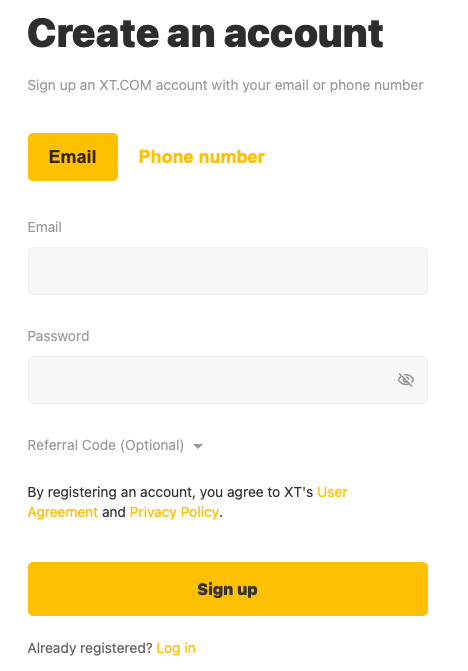The image is a screenshot of a "Create an Account" page for XT.com, prominently indicated by the large, bold black letters at the top. The background is predominantly white, and directly beneath the header, a smaller light gray text suggests, "Sign up an XT.com account with your email or phone number."

The page presents two main options for account creation: via email or phone number. 'Email' is highlighted in a black font within a yellow box, while 'Phone Number' is in black font without a box. Below these options, there are input fields with the placeholder text "Email" and "Password," both in light gray. Each field is a light gray horizontal bar; the password field is accompanied by an eye icon with a line through it, indicating the password input is hidden.

Further down, there is an optional field for a referral code, labeled in light gray text with the word "optional" in brackets. A small downward-pointing arrow suggests this is a dropdown box.

Beneath the form fields, a note in light gray states, "By registering an account, you agree to XT's user agreement and privacy policy." The phrases "user agreement" and "privacy policy" are clickable, highlighted in yellow.

At the bottom of the screenshot, a yellow horizontal rectangle spans the width of the page with the black text "Sign Up" in the center. Below this, in light gray text, "Already registered?" is placed adjacent to a yellow hyperlinked text "Log In."

The page is visually straightforward with a clean layout, guiding users seamlessly through the account creation process while ensuring key actions and links are easily accessible.